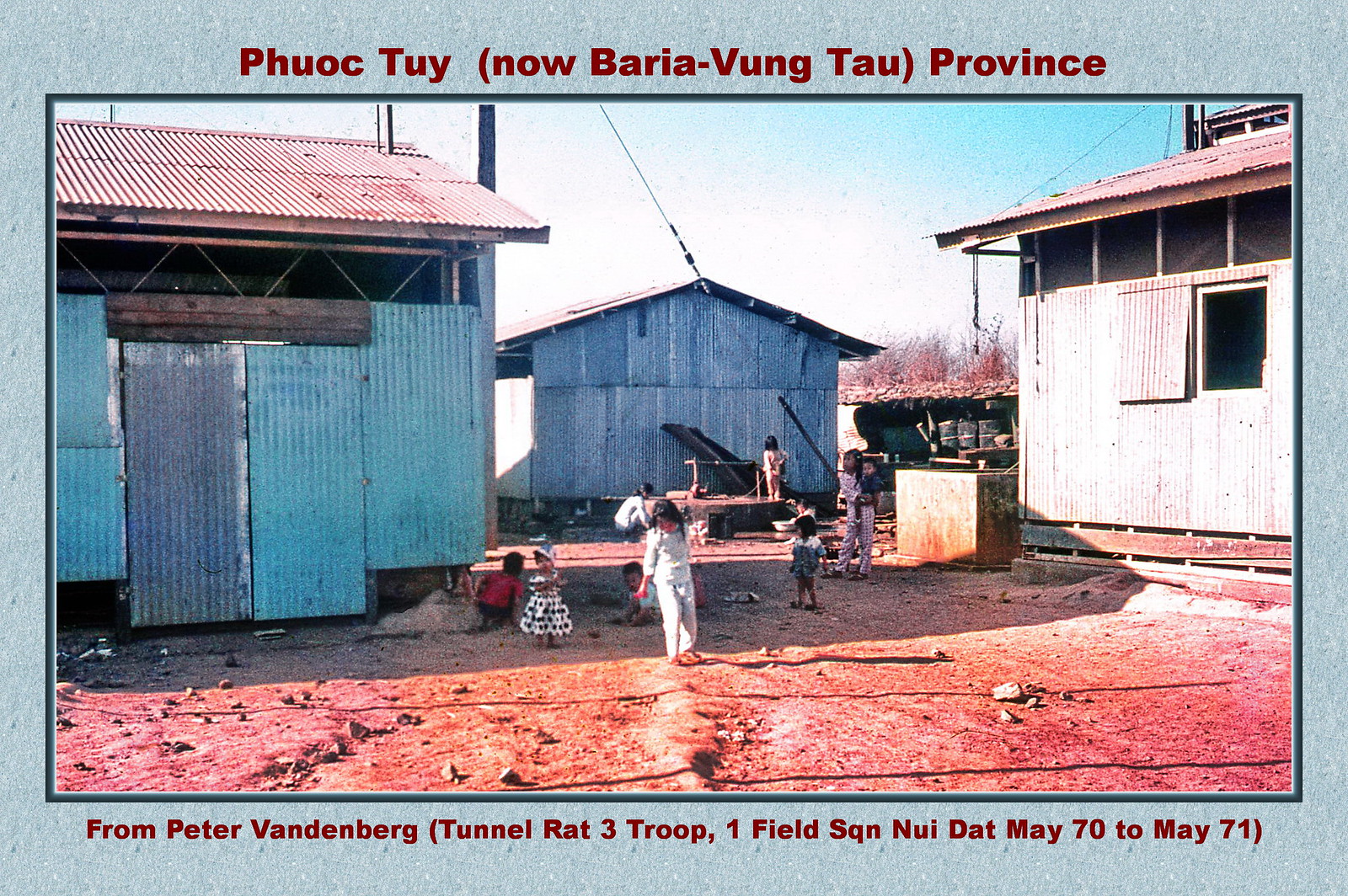This vintage landscape photograph, dating from the early 1970s, captures a scene likely in Phuoc Tuy, now known as Ba Ria-Vung Tau Province, Vietnam. The image, bordered with a blue textured frame, features black text at the top and bottom. The top inscription reads "Phuoc Tuy, Now Ba Ria-Vung Tau Province," while the bottom states, "From Peter Vandenberg, Tunnel Rat 3 Troop, 1st Field Squadron, Nui Dat May 70 to May 71."

In the foreground, around six to eight children are seen playing on a barren, brown dirt field. Some children are standing while others sit, engaged in playful activities. Surrounding the field are three makeshift buildings, constructed from corrugated metal sheets, giving a shanty-like appearance. The buildings differ in color: blue walls on the left and middle buildings, and white walls with reddish roofs on the right building. The sky backdrop is a blend of blue and white hues, enhancing the nostalgic and historical feel of the image. Additionally, cables and wires extend from the buildings, indicating possible makeshift electrical setups or construction in the area.